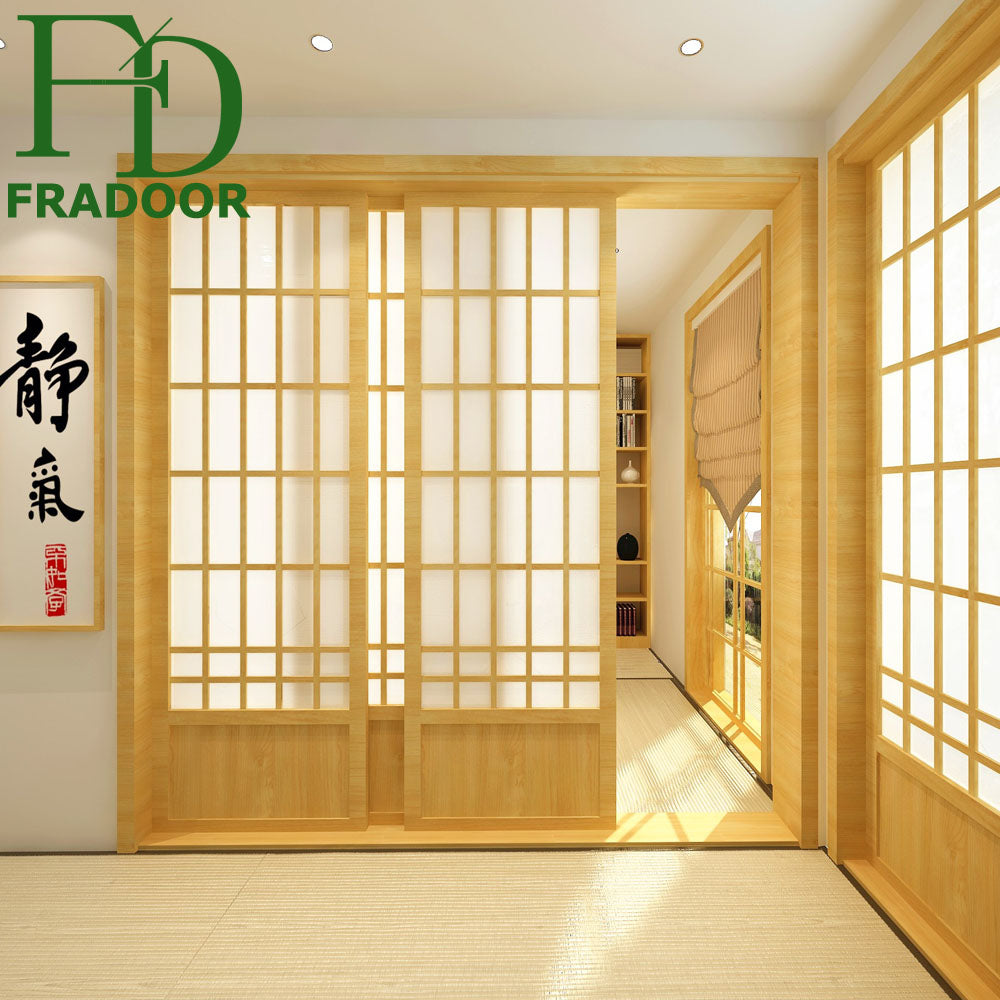This indoor photograph, perfectly square in composition, captures a tastefully decorated, Asian-themed room bathed in natural light. The floor in the foreground is a light tan wicker, extending seamlessly through a partially open sliding door, revealing a similarly styled room beyond. The sliding door, centrally featured, is constructed from light bamboo-colored wood with frosted glass panels.

The right side of the image shows a light wood wall and a window with tan wood frames arranged in rows and columns, integrating screens in their design. Through the door, the adjacent room displays a window with clear, unobstructed panes, allowing a view outside and some sunlight to filter in, casting gentle shadows over a cozy interior.

In the adjoining room, a door leads out to a patio adorned with delicate drapery. A built-in cabinet against the far wall houses various photos and decorative items, adding a personal touch to the space. A bookshelf can also be seen, holding books and a white object, enhancing the functional yet aesthetic appeal of the interior.

The left side of the image features a framed picture with black and red Chinese characters on a white background. The upper left corner of the image includes a green logo with the letters "FD" and the word "Fradoor" underneath, suggesting a brand associated with the doors or windows displayed.

Overhead, two small ceiling lights illuminate the room, complementing the natural light and warm wooden tones, creating an inviting and harmonious atmosphere.